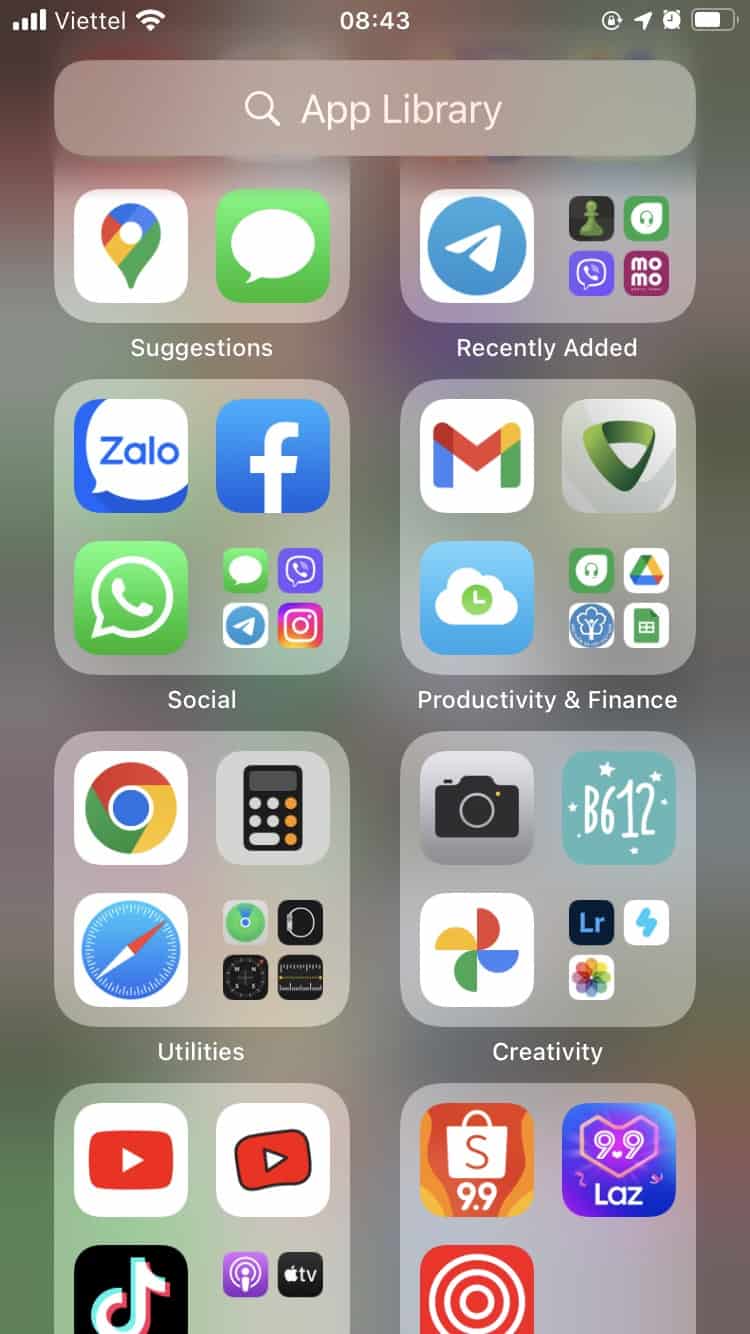A screenshot from a mobile phone displays a typical home screen layout. At the very top left corner, the cell phone reception icon is visible with the text "V-I-E-T-T-E-L" next to it, followed by the Wi-Fi reception symbol. The digital clock reads "8:43." On the upper right, the screen lock symbol, clock symbol, and battery status icon are displayed. Below this top bar is the Apple Library search bar, ready for user input.

Underneath the search bar are eight blocks representing folders, each housing various apps. The first block in the upper left corner is labeled "Suggestions," while the block to its right is titled "Recently Added." Directly below "Suggestions" is the "Social" folder, followed by the "Productivity and Finance" folder. Adjacent to "Productivity and Finance" is the "Utilities" folder, and to its right is the "Creativity" folder. The last two blocks at the bottom are partially cut off, obscuring their titles from view.